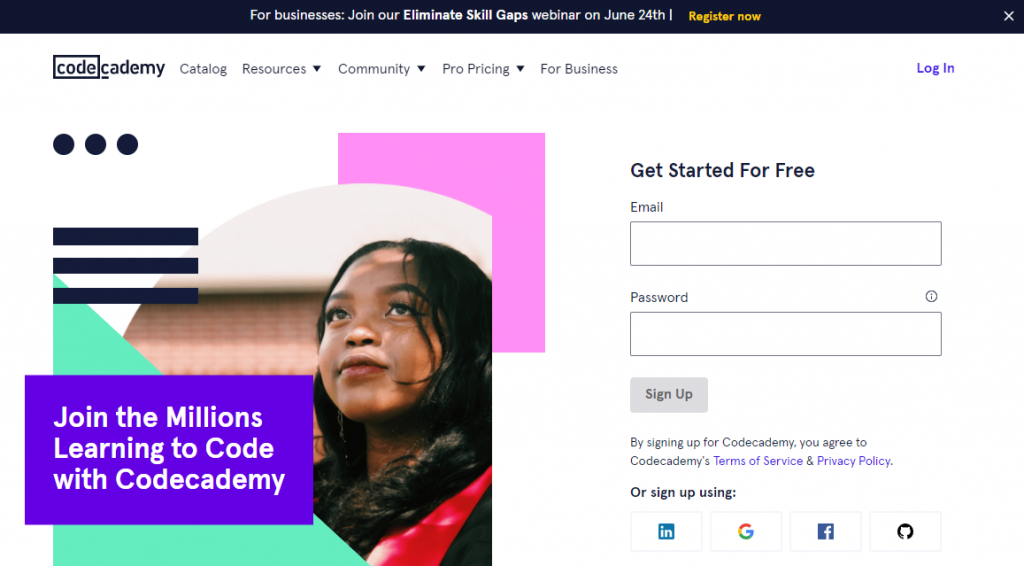Title: Comprehensive Invitation to Code Academy Webinar

Caption: The promotional image features a sleek design with a black banner at the top, announcing an upcoming webinar aimed at businesses, titled "Eliminate Skill Gaps Webinar," scheduled for June 24th. The banner includes a prominent call-to-action in yellow encouraging viewers to "Register Now." Below this, the Code Academy logo is displayed, with the word "Code" enclosed in a distinctive box. On the right side of the image, a navigational menu lists options such as "Catalog," "Resources," "Community," "Pro Pricing for Business," followed by a blue hyperlink for logging in. Further down, there's a "Get Started for Free" prompt above interactive fields for "Email" and "Password." Following these fields is a gray "Sign Up" button. An additional note clarifies that by signing up, users agree to Code Academy's Terms of Service and Privacy Policy, with alternative sign-up options via LinkedIn, Google, and Facebook also provided. The left side of the image highlights a striking blue rectangle with the message, "Join the millions learning to code with Code Academy," set against a vibrant teal and purple gradient background.